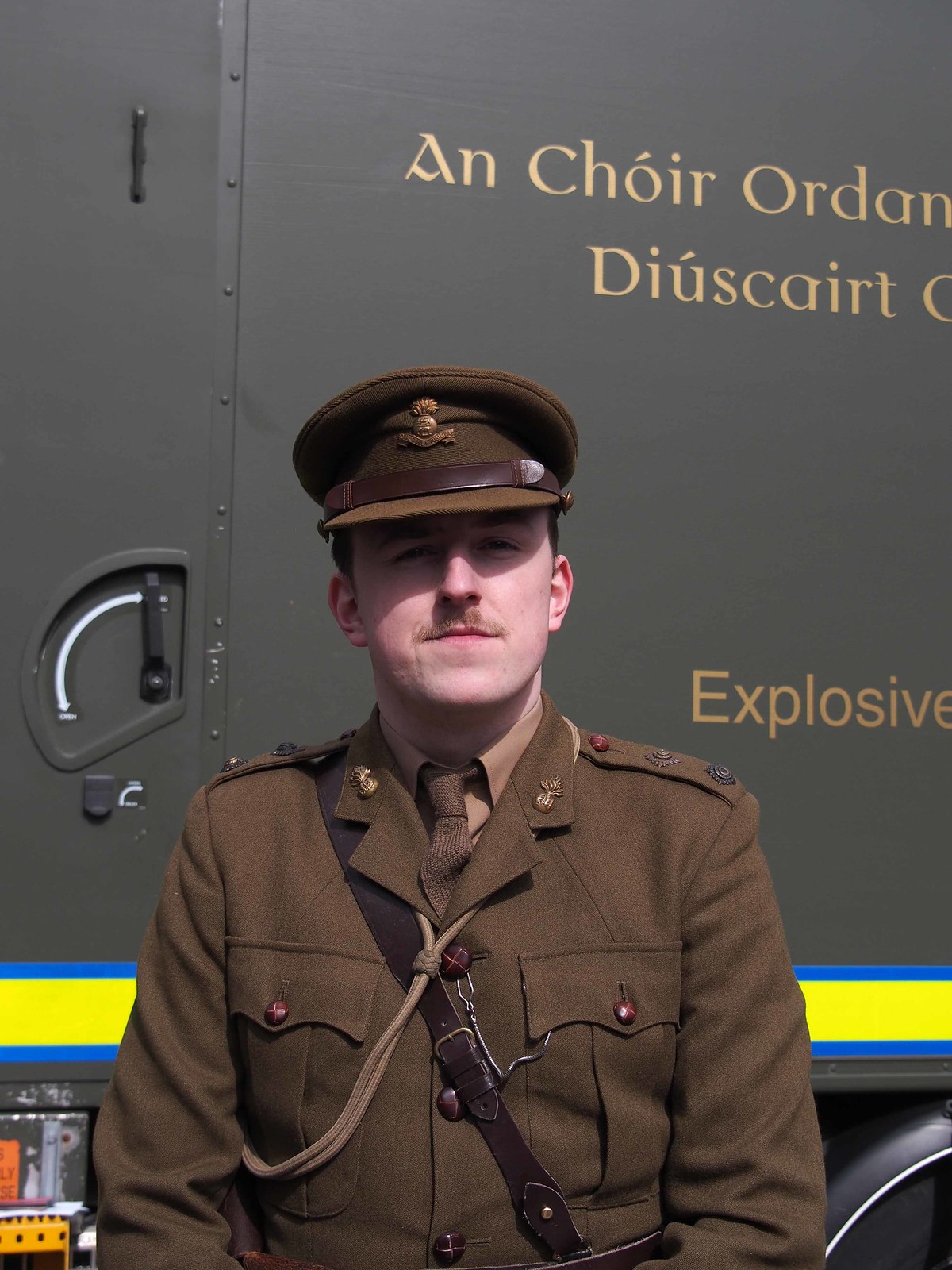The photograph depicts a stern-looking soldier in a brown uniform and a matching brown hat, adorned with a metal pin on the front and casting a distinct shadow over his light-complected, slightly reddish face. His eyebrows frame narrow eyes, and he sports a light brown mustache. The soldier's heavy, olive-brown jacket, buttoned up with a rope tie around the collar, partially reveals a lighter brown shirt underneath and a dark tie. Across his chest, a decorative rope and a sash are visible, and a sling is draped over his shoulder. The image is cropped to show him from the head down to his elbows.

Behind the soldier, there is a green metal bin or truck with multiple inscriptions in a foreign language, partially visible and including the words "explosive." The green surface features a prominent fluorescent yellow stripe, bordered by blue stripes on both the top and bottom, and a white arrow indicating how to open a latch. The bright daylight emphasizes the sharp shadow of his hat across his face and enhances the clarity of the detailed surroundings.